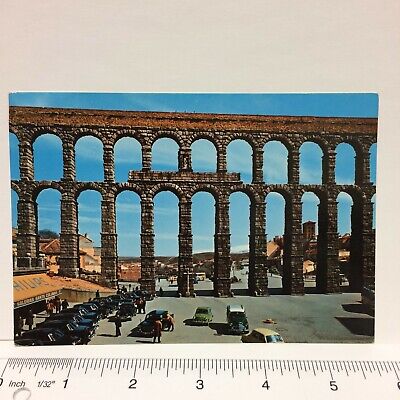This image is a photograph of an ancient Roman aqueduct, captured in what appears to be a vintage print, likely from the mid-20th century. The aqueduct, a majestic stone structure, stands impressively tall, around eight stories high, dwarfing the surrounding buildings. It features two distinct stories of arches—elongated ones on the lower level and shorter ones on top—with a straight plinth crowning the structure. The material comprises gray stones stacked meticulously with a brownish plinth atop.

In the foreground, a parking lot with vintage cars, including black, green, and yellow models from the 40s and 50s, rests on a gray surface. The scene is set against a beautiful blue sky, dotted with some clouds. Surrounding the aqueduct are sand-colored and brown stone buildings, framed by distant mountains, indicating a picturesque setting, likely in Italy. The photograph, slightly shy of six inches wide as indicated by a white ruler lying next to it on a grayish-tan background, suggests the image might also be a postcard, emphasizing its historical and aesthetic charm.